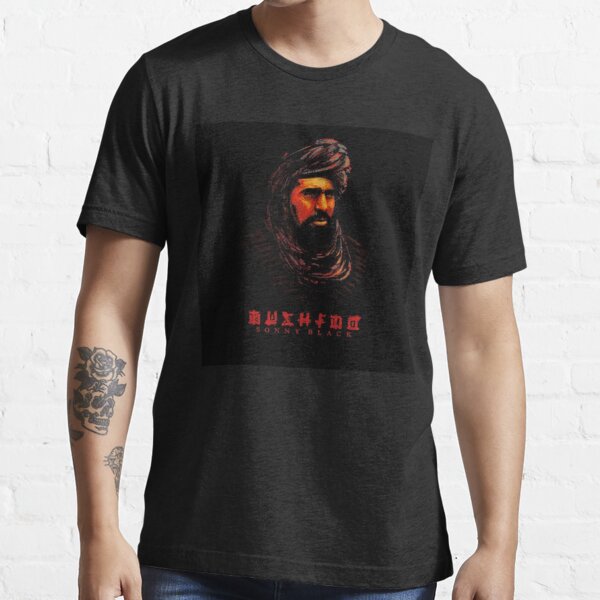This is a slightly blurry photograph capturing a man from the neck down to just above his crotch, against a white brick wall. He is wearing a dark chocolate brown t-shirt with a darker brown square graphic on the front. The graphic features an image of an Arab man, highlighted with lighter tan folds in his dark brown turban, looking to his left (the right side of the image). The man in the graphic has a black beard and black mustache, and beneath him, there is partially legible red text that appears to say "BWI HIDE" in block printing. The man in the photograph has bare arms with a prominent rose tattoo, partially obscured by his elbow, on his right forearm. He stands front and center, and the image is taken with studio lighting which casts a stark contrast against the washed-out white brick wall behind him.